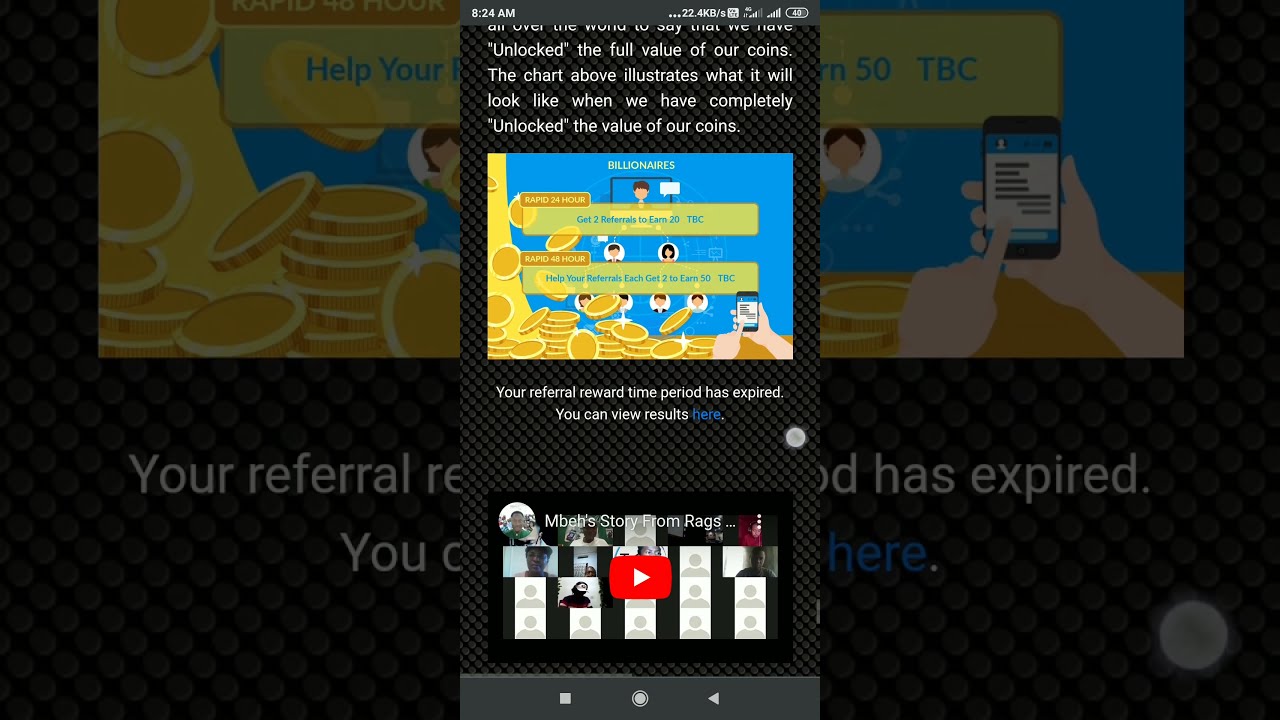This screenshot, likely from an economic learning game or app, features a central blue, yellow, and brown-themed interface. The key message displayed is "Economy from the ground up: the full value of these coins are locked up until we have enough merchants spread all over the world to say that we have unlocked the full value of our coins." Above this, there's a chart illustrating the potential unlocked value of the coins. Gold coins are prominently featured throughout the image, with labels such as "rapid 24 hours" and "rapid 48 hours," and "50 TBC," suggesting mechanisms for potential earnings. The lower section notes, "Your referral reward time period has expired. You can view your results here," on a black background. A cartoon hand holding a phone appears in the lower right corner, emphasizing the app's accessibility. Additionally, the top of the screenshot displays "8:23 AM" along with the Wi-Fi signal, indicating it’s a live mobile app interface.